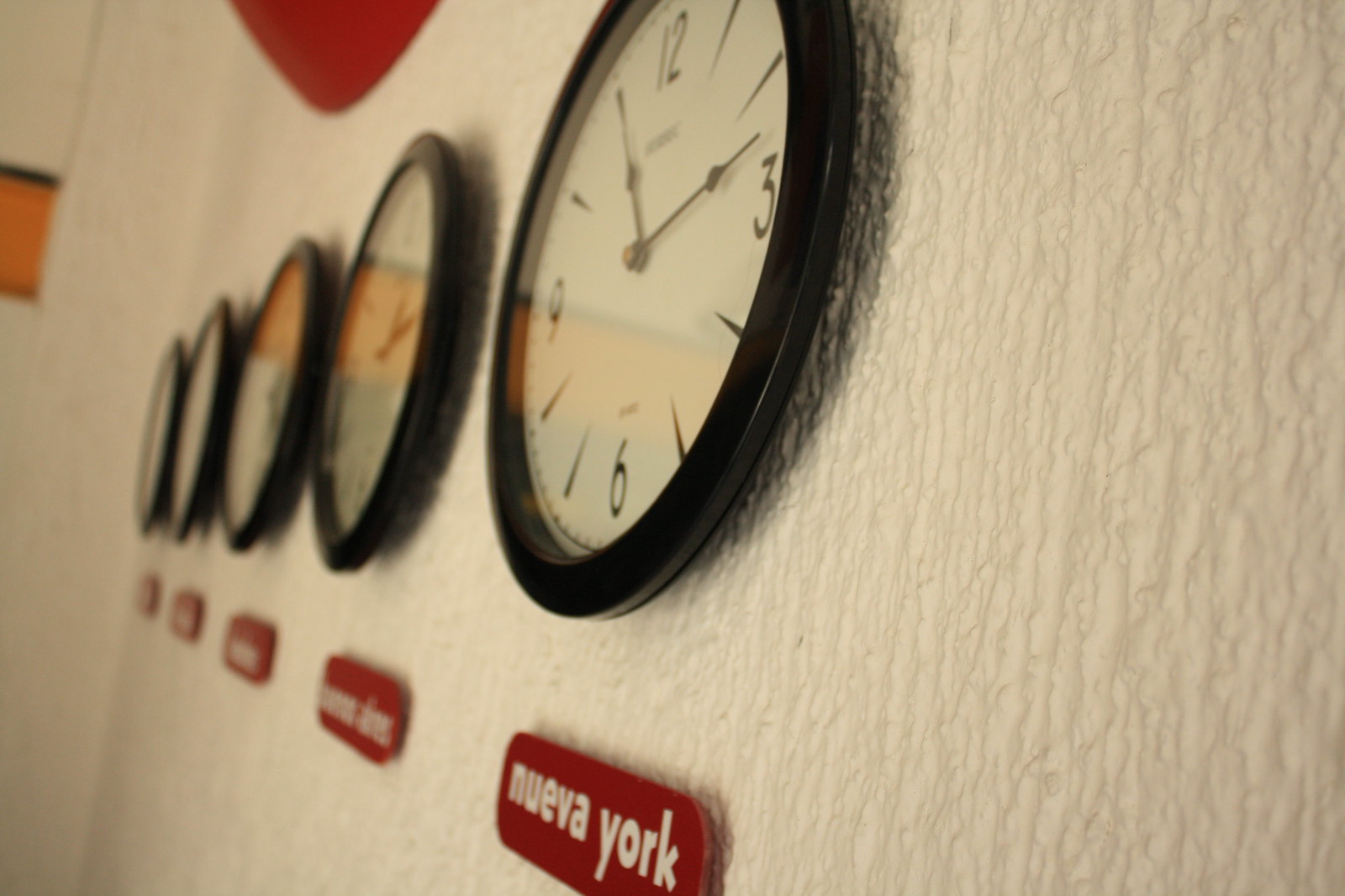The image showcases five black clocks, each labeled with different time zones. The clocks have a minimalist design featuring white faces with black numerals and hands. The visible clock, labeled "Nuevo York," suggests it displays the time for New York. The variety of time zones indicates a global context, likely in an international setting. The clocks are mounted on a plain, off-white wall, which adds a stark contrast to their black frames, emphasizing their functional simplicity.